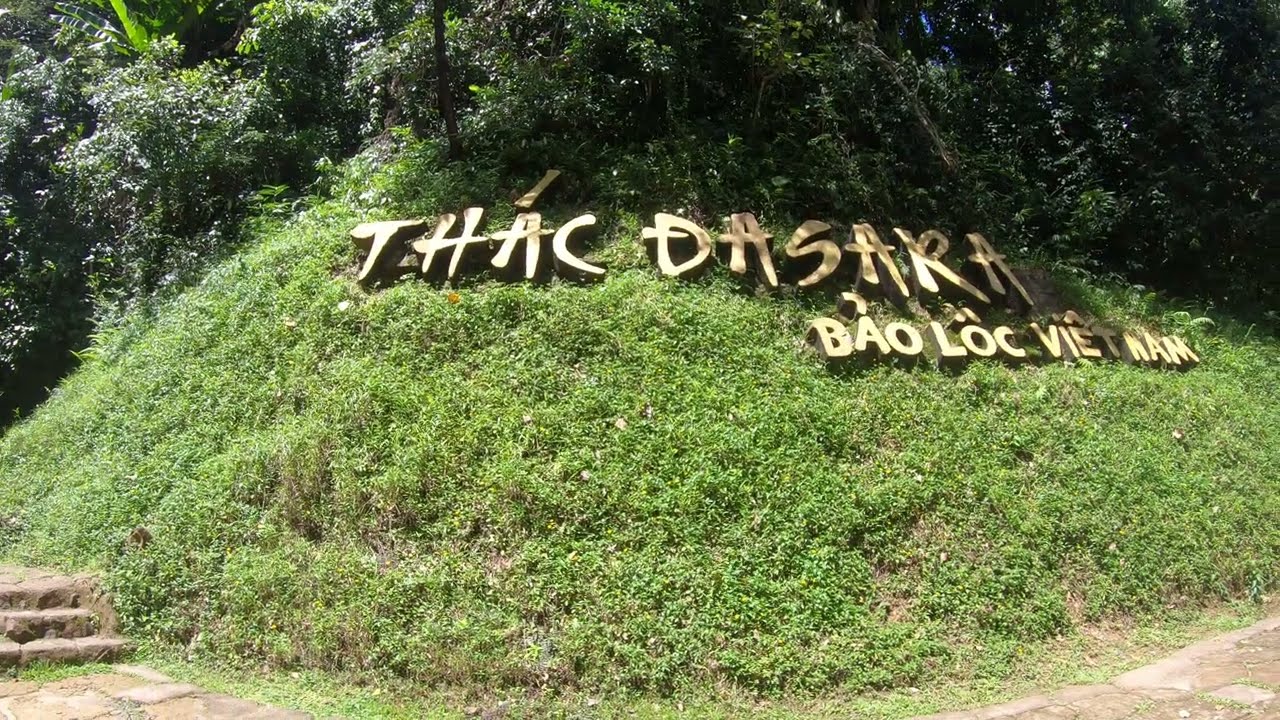The image is a brightly lit outdoor scene taken on a sunny day, showcasing a steep grassy hill adorned with large wooden letters that spell out "THAC DASARA" and "BAO LOC, VIETNAM." The top of the hill is populated with large bushes and numerous green trees, creating a dense natural backdrop. In the bottom right corner of the photo, a stone brick pathway curves around the hill, leading to three cement steps ascending to the left. The entire scene suggests an inviting, nature-centric area, possibly a park, where visitors can enjoy the lush surroundings and scenic views.